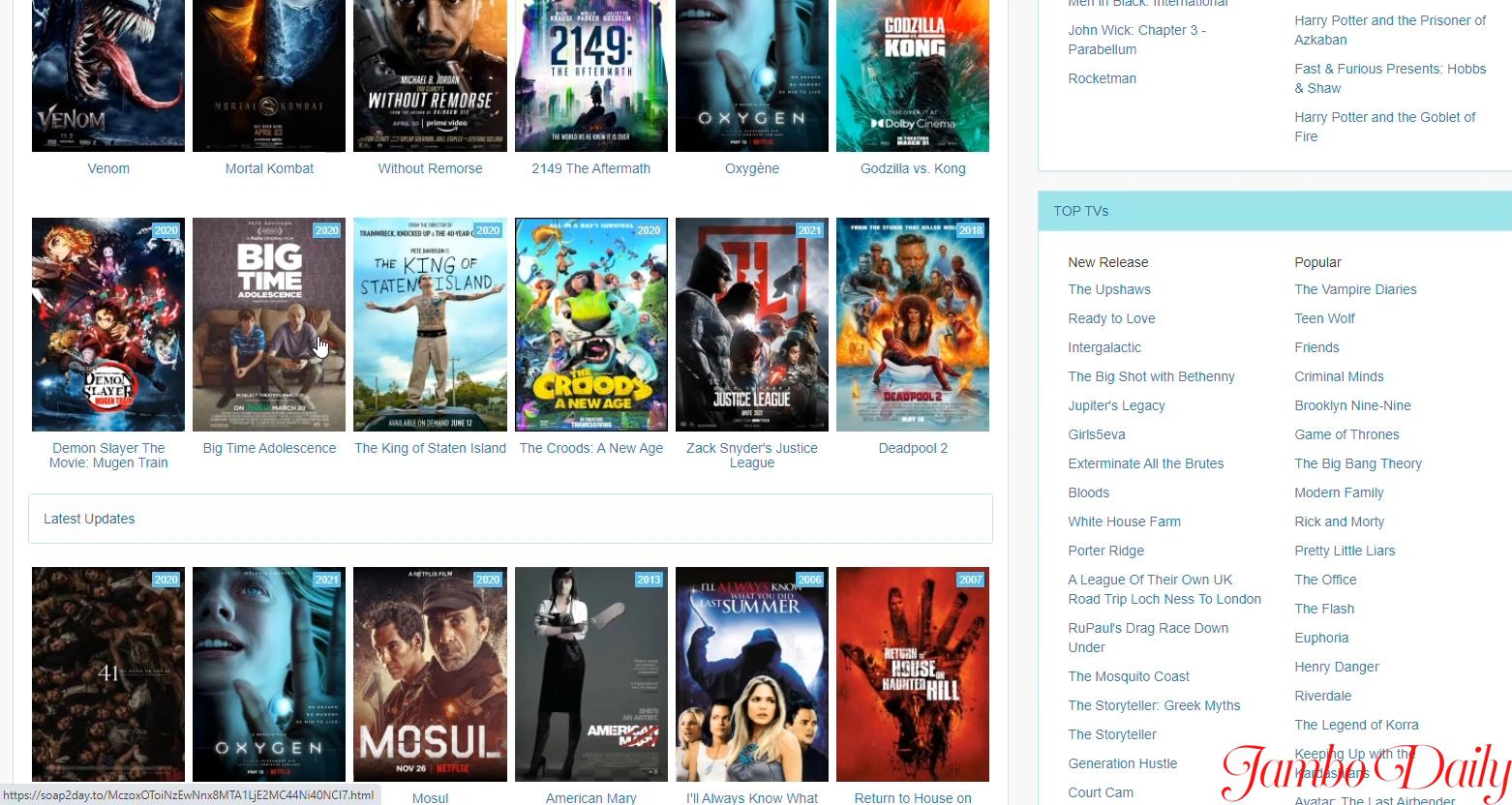A meticulously cropped screenshot from the website **soap2day.to**, featuring a curated selection of movie advertisement covers and TV listings. In the bottom left-hand corner, the website URL is subtly visible, while the bottom right-hand corner bears a bold red watermark reading "Jambo Daily." 

On the left side of the image, 18 small, thumbnail-style icons showcase movies with their titles prominently displayed underneath in blue text. These movies include popular titles such as *Godzilla vs. Kong*, *Demon Slayer*, and *Venom*.

Adjacent to the movie thumbnails, on the left-hand side, a neat box presents information in two columns: one listing new TV releases and the other highlighting popular TV shows.